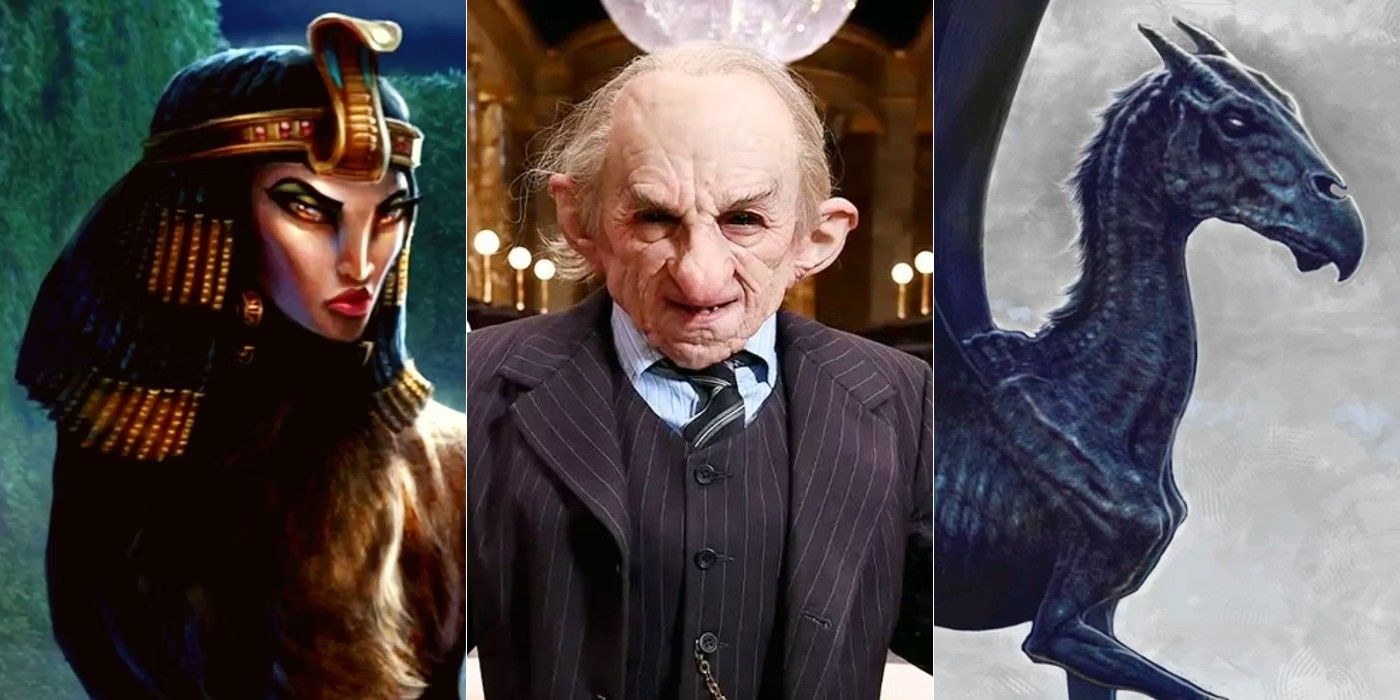This image is a detailed collage divided into three distinct sections. The left third portrays an Egyptian-looking woman, possibly resembling a sphinx or Medusa, with an intricately adorned snake headband and dreadlock-style hair threaded with golden beads. Her face, possessing classic Egyptian features with angry eyes and red lips, is set against a dark blue night sky and a lush forest backdrop. The middle third features a very old, goblin-like man with a heavily wrinkled face, large nose, and sparse, wildly outstretched hair. Dressed in a suit and tie, he stands under a chandelier-like light, with circular lights behind him suggesting the interior of a grand building. The right third shows a dark navy blue to black skeletal, dragon-like creature with horns, reminiscent of a pterodactyl or a horse. This creature is set against a crystalline white background, possibly suggesting a moonlit night.